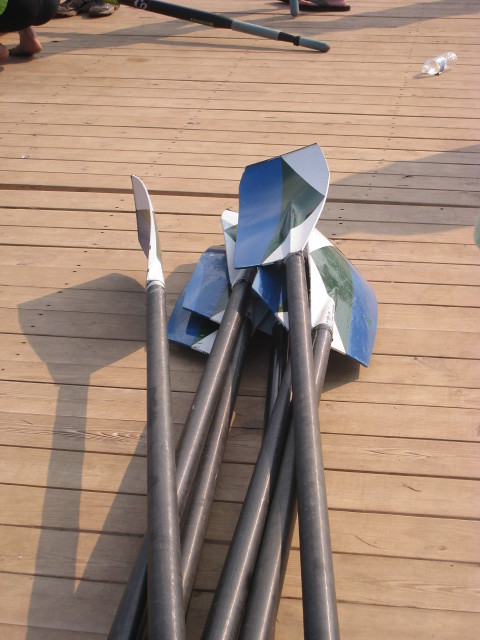The photograph depicts six oars stacked in a pile on a horizontal wooden deck. The deck is detailed with visible wood grain, knotting, and the marks of nails or screws where the planks are affixed to the supports. The oar handles are a dark gray, almost black color. The blades feature a striking design with colors that transition from blue to green, and culminate in two white triangles. The blades have a shape reminiscent of shovels. In the top right corner of the frame, there is a clear, empty plastic water bottle lying on its side. The top left corner shows part of a human foot and an object that might be another oar. The scene is set on what appears to be a dock, characterized by its regular, natural wood color.